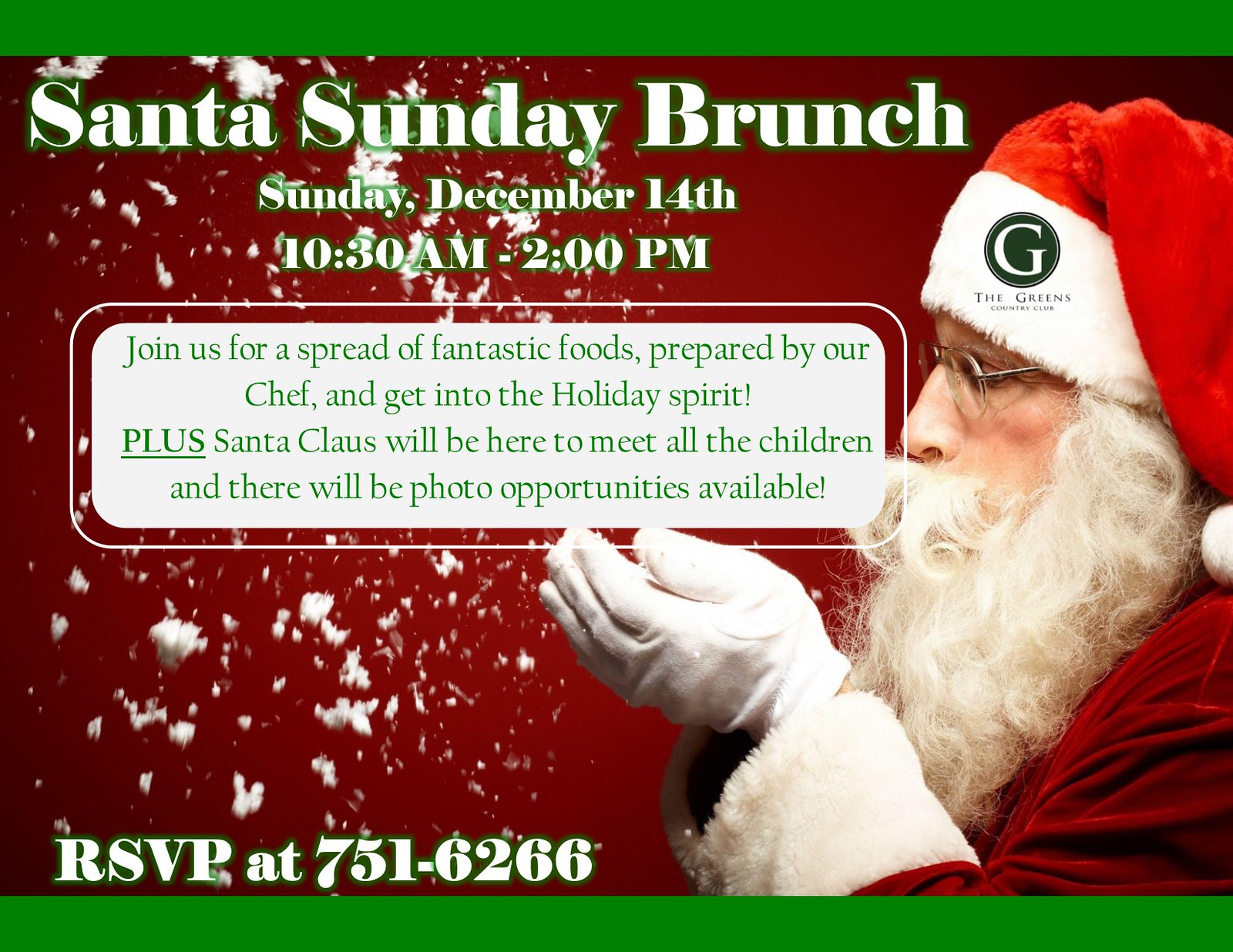The image is an event poster for a "Santa Sunday Brunch." The poster features a green border at the top and bottom, with a bright red background. Positioned on the right side of the poster, Santa Claus is depicted blowing snow from his cupped hands. He is adorned in his classic red hat with a white pom-pom, glasses, a fluffy white beard, white gloves, and a red coat with fluffy white cuffs. 

At the top, the poster announces in large, white letters: "Santa Sunday Brunch, Sunday, December 14th, 10:30 a.m. to 2:00 p.m." Beneath this, in green font on a white rectangle background, it invites attendees to "join us for a spread of fantastic foods prepared by our chef and get into the holiday spirit. Plus, Santa Claus will be here to meet all the children and there will be photo opportunities available."

At the bottom in white letters, the poster requests RSVPs at the phone number 751-6266. Additionally, Santa's red hat features "The Greens Country Club" embroidered on the white cuff, alongside a logo consisting of a white letter "G" inside a dark green circle.